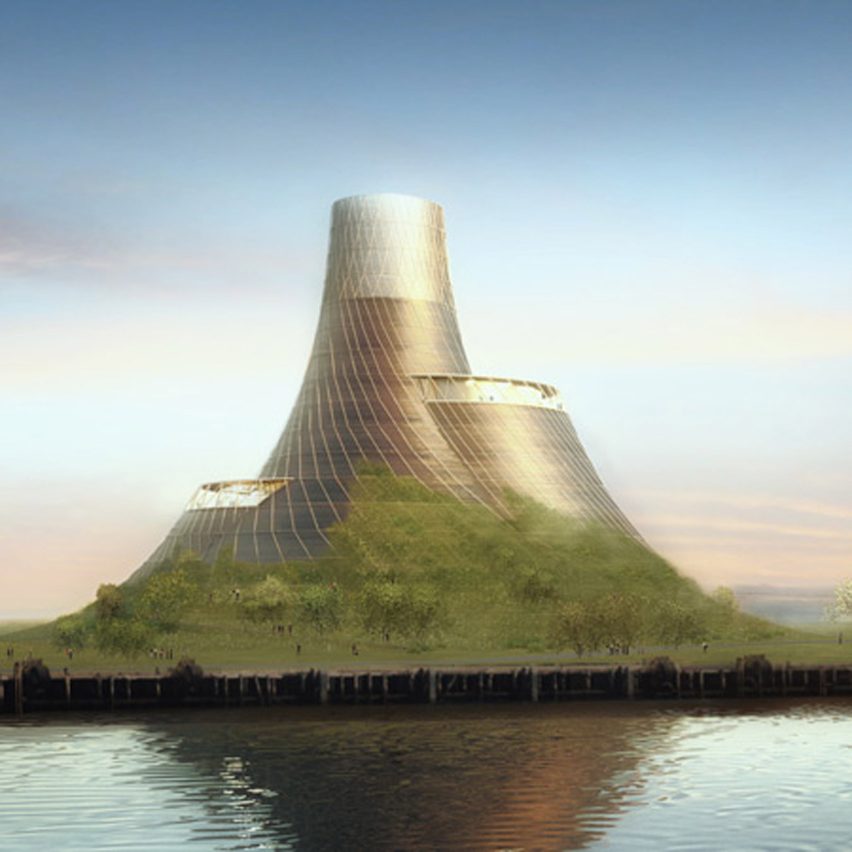This image depicts a striking, futuristic structure on a verdant island, surrounded by a shimmering expanse of water. Central to the scene is a large, metallic, cone-shaped building that evokes the form of a nuclear reactor yet diverges with its unique, industrial design. The main structure features spiraling, arcing lines reaching to its apex and has staggered attachments on either side, creating an almost mountainous silhouette. Encircling the primary form are smaller buildings, some adorned with windows. The edifice seamlessly transitions into the lush greenery of the island, where small, indistinct figures appear to be walking. Above, the sky is tinged with pink hues, suggesting a sunrise or sunset, and there is a brilliant flash of white light, perhaps from the sun reflecting off the metallic surfaces. The overall composition, with its blend of natural and industrial elements and the sharp contrasts between them, hints at an AI-generated origin.